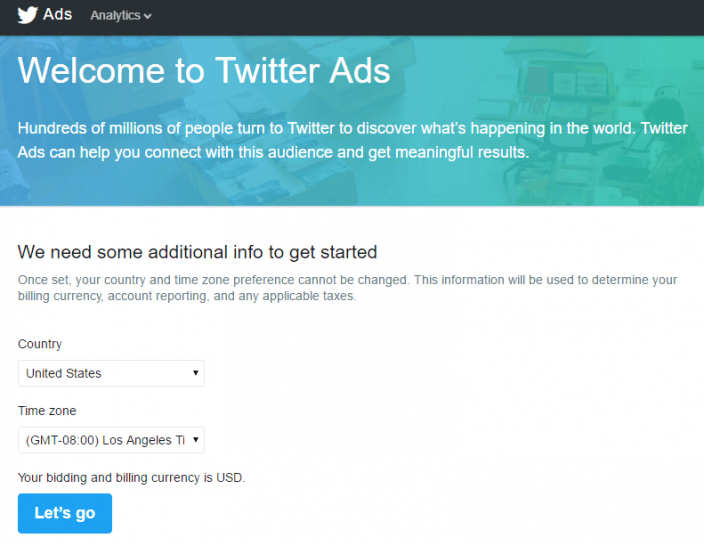Screenshot of a Twitter Ads Web Page

The image is a screenshot of a Twitter webpage dedicated to Twitter Ads. The top portion of the page features a black banner with the Twitter logo on the left, followed by the word "Ads" and a scroll-down section labeled "Analytics." Directly below this is a visually appealing banner with a blue-aqua gradient flowing from left to right, overlaying a softly focused image of people working. The banner displays the text: "Welcome to Twitter Ads. Hundreds of millions of people turn to Twitter to discover what's happening in the world. Twitter ads can help you connect with this audience and get meaningful results."

Below this colorful banner is a section with the message: "We need some additional info to get started." Additional text provides further instructions on the required information. On the left side, there are drop-down menus for selecting country and time zone. The country drop-down menu has "United States" selected, and the time zone drop-down menu is set to "GMT-8 Los Angeles time." Below these selections, the text reads: "Your bidding and billing currency is USD." At the lower left corner is a prominent "Let's Go" button. 

The bottom part of the page features a clean, solid white background with ample empty space, giving it an uncluttered appearance. There is no visible border outlining this section.